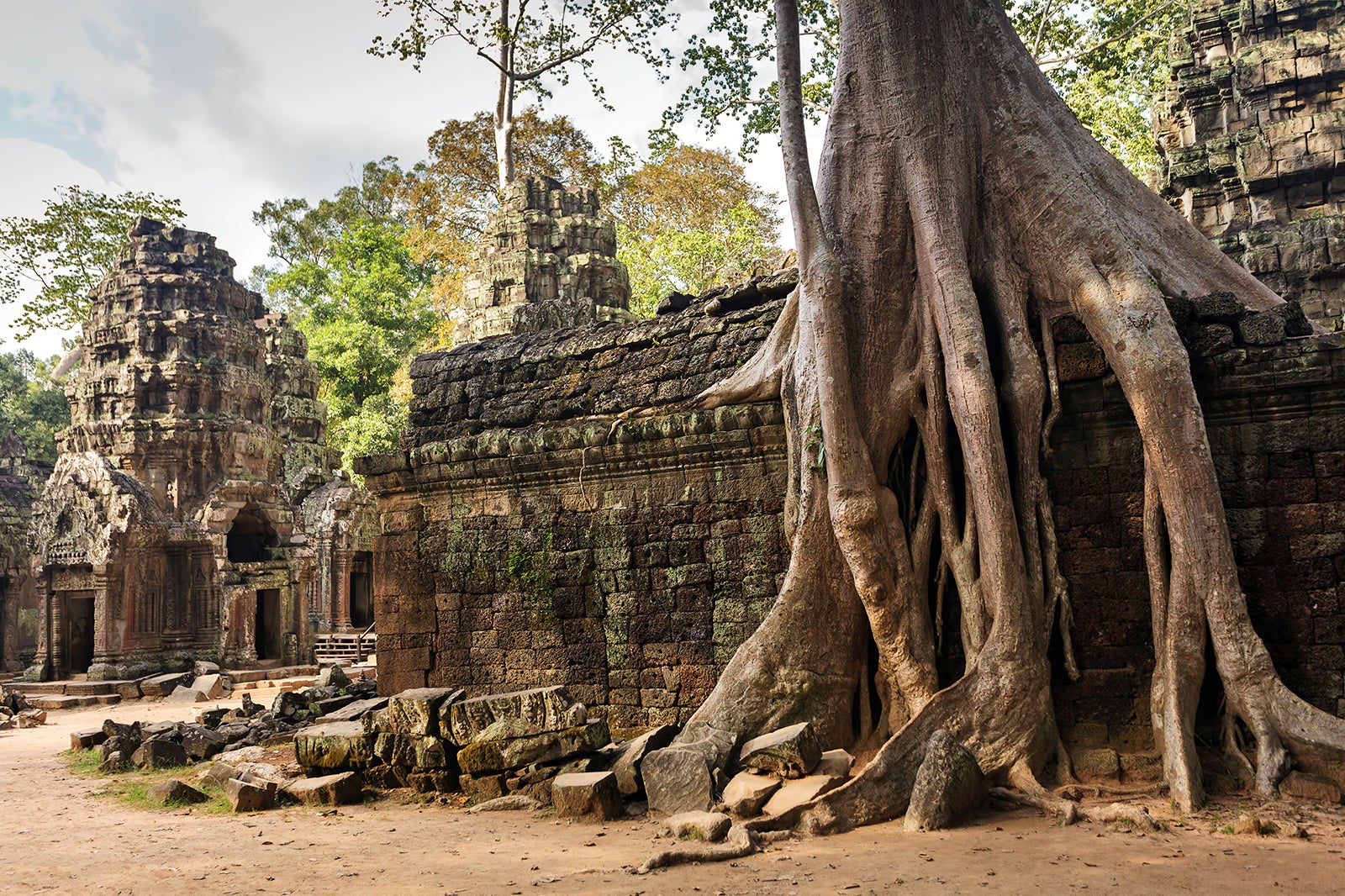This image depicts a wide-angle, photorealistic scene of an overgrown ancient ruin, reminiscent of a Cambodian temple in the Angkor Wat style. Central to the image is a weathered sandstone temple, characterized by intricate details above a crumbling doorway and a colossal tree whose roots cascade dramatically over the temple walls, reaching down to the ground. Surrounding the main structure are scattered, broken building blocks, contributing to the sense of decay. In the background, additional ruined tower buildings rise amidst a thick canopy of jungle trees, with the overcast, gray sky accentuating the ancient, mysterious atmosphere. The sandy walkway winding through the complex evokes the temple's historical and cultural depth.